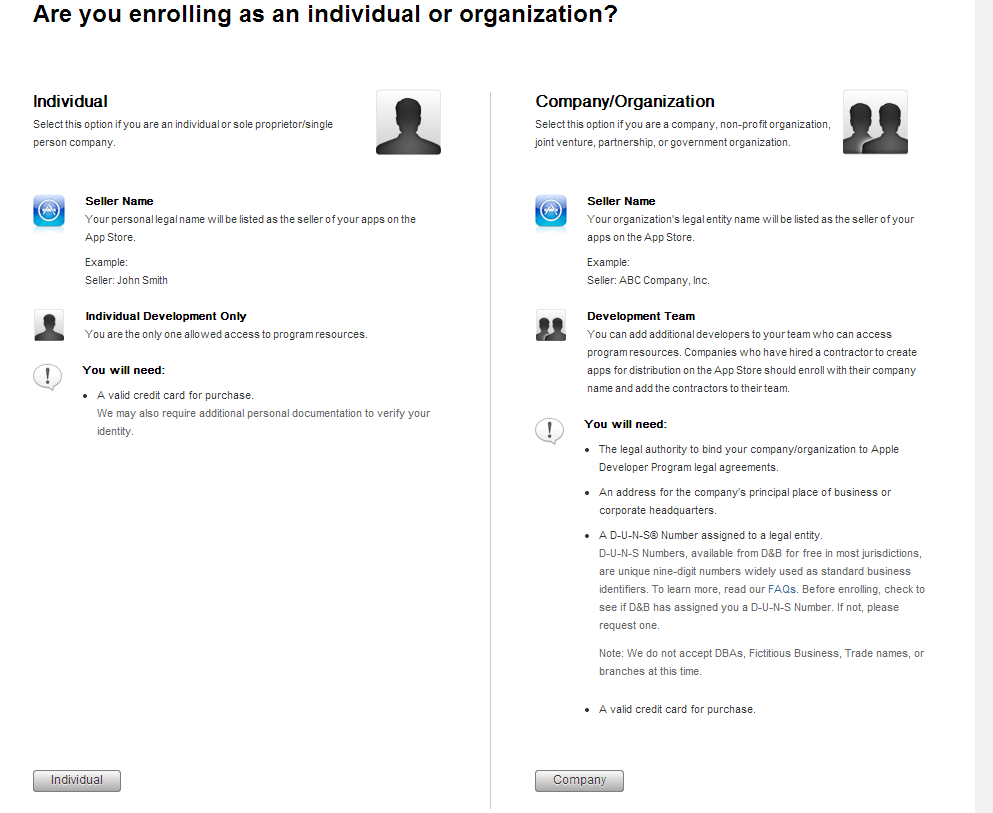The image depicts a split-screen layout with a gray vertical line dividing the content into two sections. At the top of the image, a prompt in black text reads: "Are you enrolling as an individual or an organization?"

**Left Section: Individual Enrollment**
- Heading: "Individual"
- Description: "Select this option if you're an individual or sole proprietor/single-person company."
- Details:
  - **Seller Name:** "Your personal legal name will be listed as the seller of your apps on the App Store. For example, 'Seller John Smith'."
  - **Individual Development Only:** "You are the only one allowed access to this program's resources."
  - **Requirements:** "You will need a valid credit card for purchase. Additional personal documentation may be required to verify your identity."

**Right Section: Company/Organization Enrollment**
- Heading: "Company/Organization"
- Description: "Select this option if you are a company, non-profit organization, joint venture, partnership, or government organization."
- Details:
  - **Seller's Name:** "Your organization's legal entity name will be listed as the seller of your apps on the App Store. For example, 'Seller ABC Company Incorporated'."
  - **Development Team:** "You can add additional developers to your team who can access program resources. Companies that have hired a contractor to create apps for distribution on the App Store should enroll with their company's name and add the contractor to their team."
  - **Requirements:** "You will need the legal authority to enroll."

The overall visual presentation clearly delineates the enrollment options and provides comprehensive details on the requirements and benefits for both individual and organizational enrollment in the program.